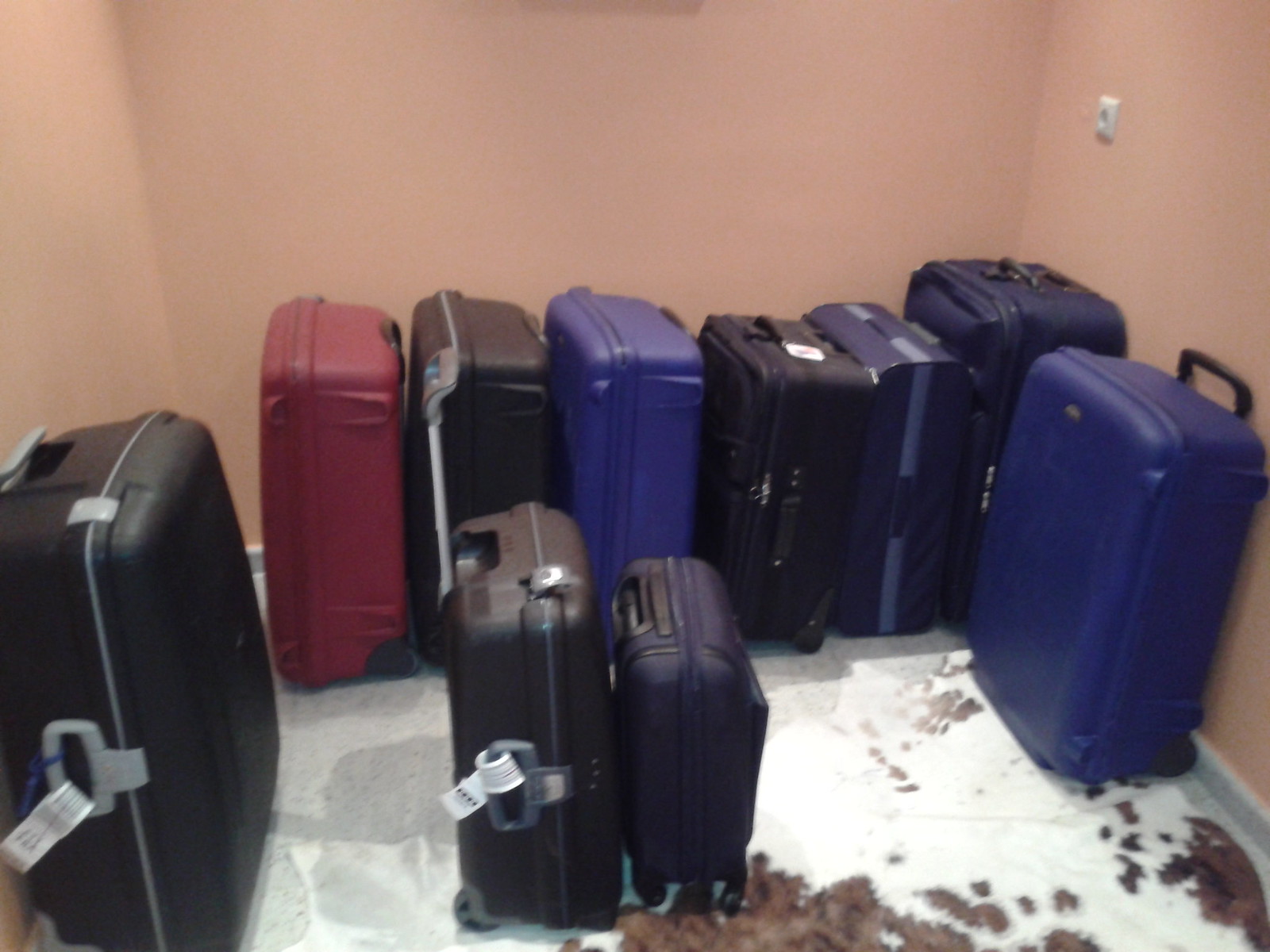The image captures a cluttered room with tan or peach-colored walls, filled with various pieces of luggage. The floor features a distinctive white cowhide rug with brown spots, contrasting against the white floor beneath it. A diverse assortment of suitcases is scattered throughout the room; these include both check-in and carry-on types, made from materials ranging from hard shell to nylon, and varying in colors such as blue, black, and red.

Approximately ten suitcases are arranged in the space. Six of them are lined up against the wall; among these, a noticeable blue suitcase leans against one side of the wall, while another larger suitcase stands at the opposite end. In the center of the room, two more suitcases stand upright. Some of the luggage bears airplane tags, suggesting recent travel, while others remain untagged. The overall scene conveys a sense of organized chaos within a modestly decorated interior.